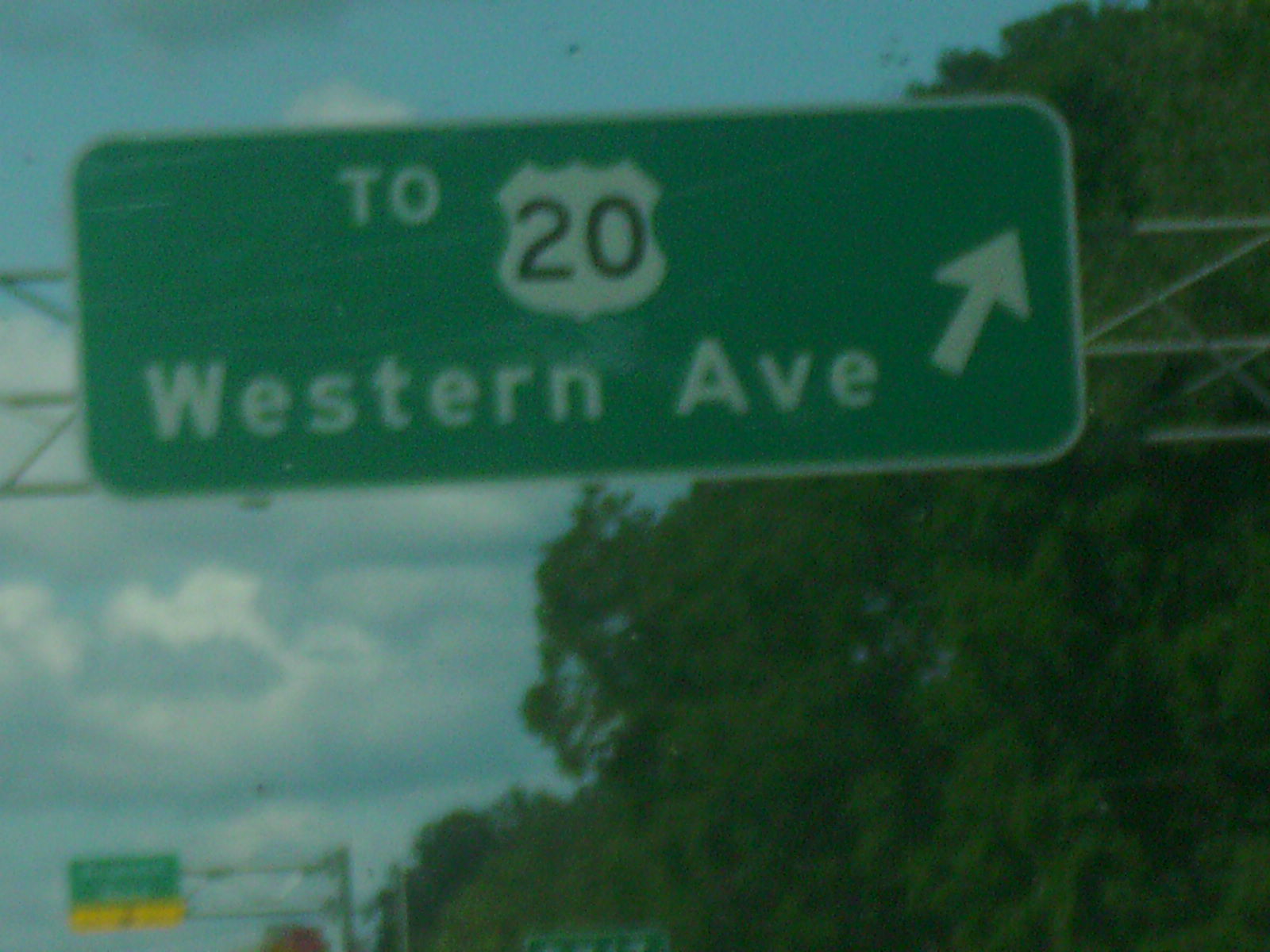The photograph captures an overhead view of a green rectangular highway sign taken from a moving vehicle. The sign, framed with white reflective paint, reads "220 Western Avenue" with an arrow pointing diagonally to the right. The sign is supported by a skeletal silver metal structure that spans above the road. In the background, there is another highway sign, also green with a touch of yellow at the bottom, though its details are not legible. The scene features the blue sky scattered with white clouds and several trees visible primarily to the right. A large green bush is also present behind the primary road sign towards the right side. This image appears to be oriented on an expressway, captured from a perspective just above the road, emphasizing the signage and scenic elements rather than the vehicles.